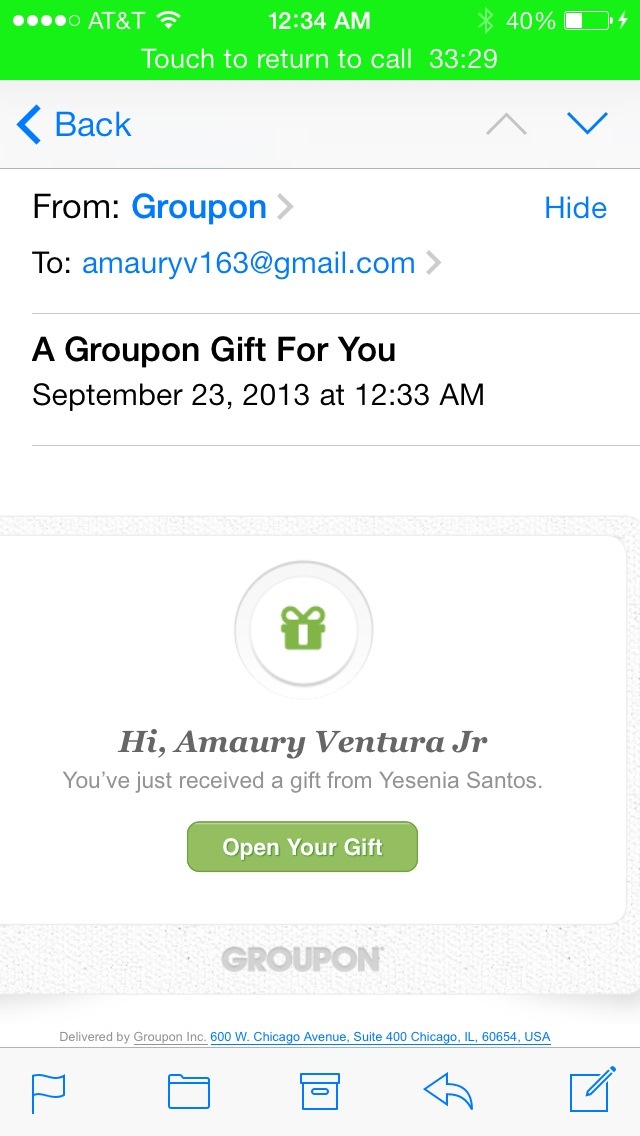The image is a screenshot of a vertically oriented smartphone screen, displaying an email from Groupon. At the top, there is a bright yellow bar indicating phone details such as the network provider (AT&T), connection type, call status (active for 33 minutes and 29 seconds), time (12:34 a.m.), and battery percentage (40%). Immediately below this bar is the phone interface indicating a "touch to return to call" option. 

The email interface follows, showing the sender as Groupon and the recipient as amoriv163@gmail.com. The subject line reads, "A Groupon gift for you," dated September 23rd, 2013 at 12:33 a.m. The body of the email includes a green silhouette of a present, accompanied by the text, "Hi Amori Ventura Jr., you've just received a gift from Yesenia Santos." Below this message is a prominent blue banner with the inscription "Open your gift." The email footer features the Groupon logo and a series of icons at the very bottom, which include a flag, file folder, file box, arrow, and pencil on a notepad, indicating various possible actions.